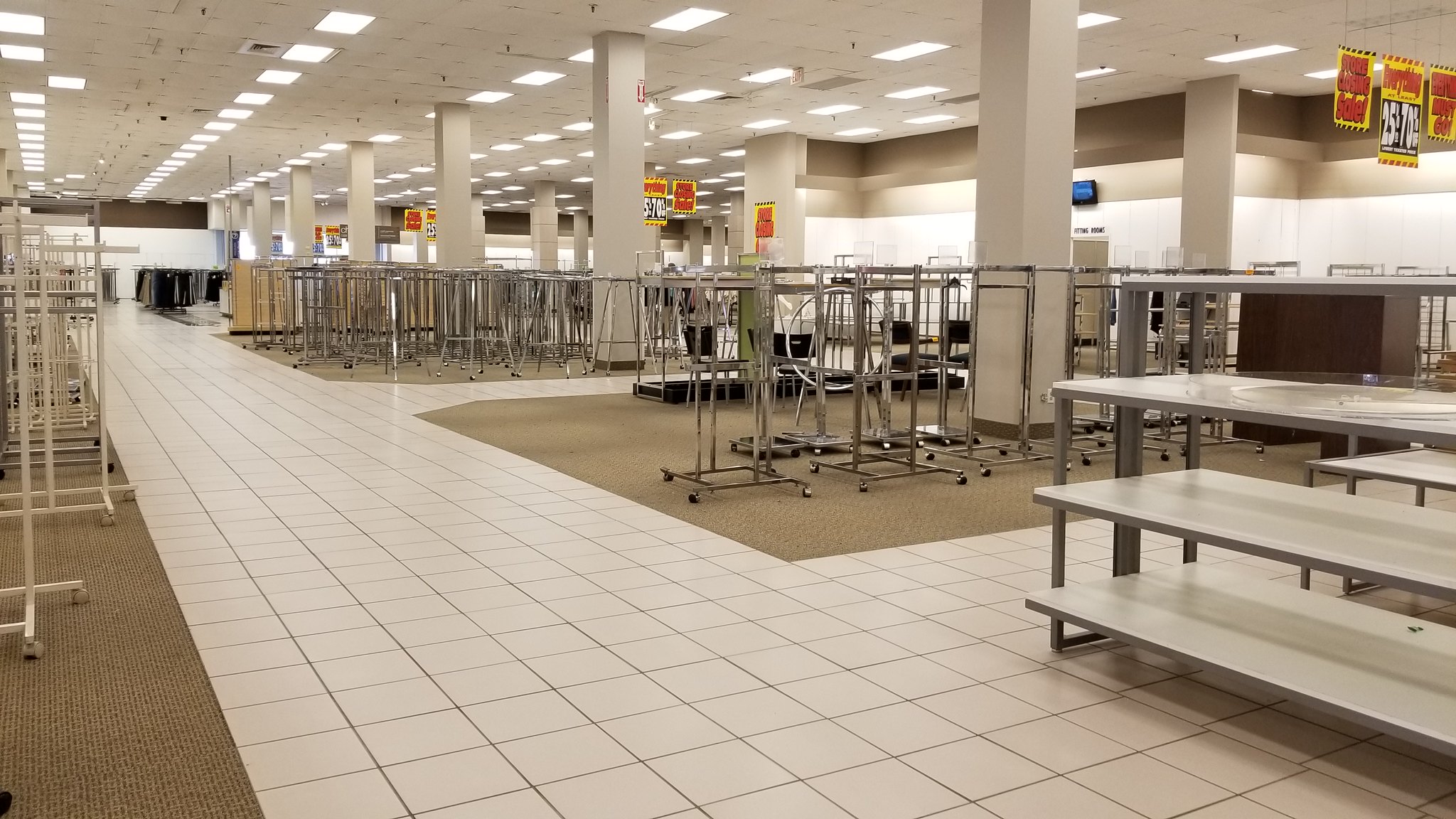This image captures a desolate interior of the K-Mart in Parma, Ohio, which has recently gone out of business. The photograph, taken from an angle, reveals an empty department store with barren clothes racks and shelves dispersed across the space. Dominating the center is a white tiled walkway that loops around the store and leads to carpeted sections where specific products once resided. On the left corner, the tightly woven brown carpet contrasts with the central tile flooring. The ceiling is lined with numerous fluorescent light tiles, casting a stark, uniform glow over the scene. Hanging from the ceiling are red and yellow signs announcing the store’s closure and advertising discounts ranging from 25% to 70% off. Though most shelves and racks are devoid of merchandise, a few racks in the distance, particularly on the upper left side, still hold some clothing items such as jeans and sweatpants. This bleak image poignantly illustrates the final days of the once-bustling K-Mart.